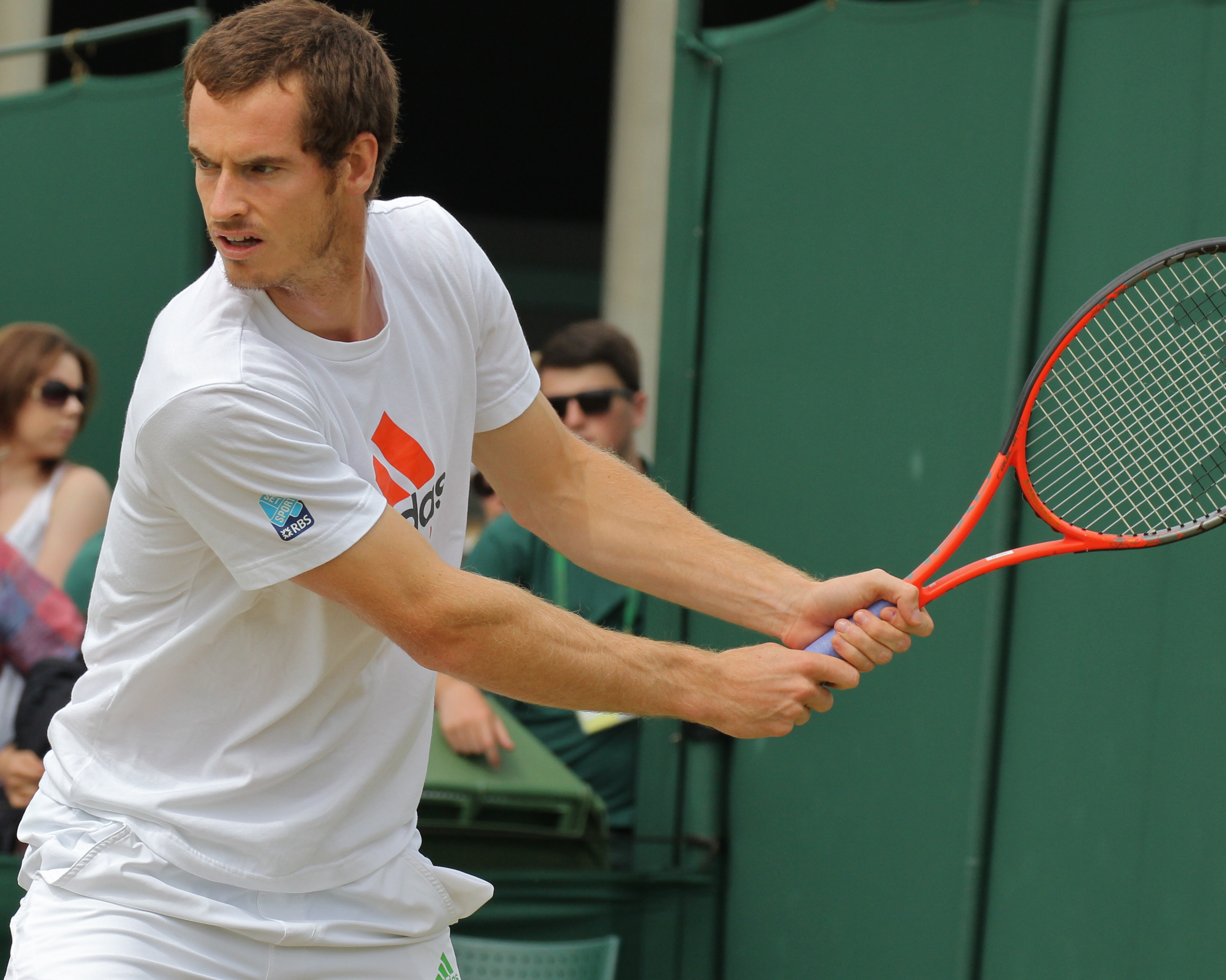This is a detailed photograph taken in a sports complex, capturing a tennis player mid-game. The player, a man with short brown hair, is wearing a white, half-sleeve t-shirt adorned with the Adidas logo in black, accompanied by red stripes, and paired with white shorts. He stands with his body facing the right while his head turns to the left, focusing intently. In his hands, he grips a red tennis racket with a blue grip, seemingly in the action of attempting to hit an unseen tennis ball. 

In the background, the scene includes several spectators. Prominently, two individuals stand out among the watchers: a short brown-haired woman wearing sunglasses positioned on the far left and a man also wearing sunglasses situated a bit to her right. Surrounding these spectators, dark green portable mats and other background elements imply the setting's sporting environment.